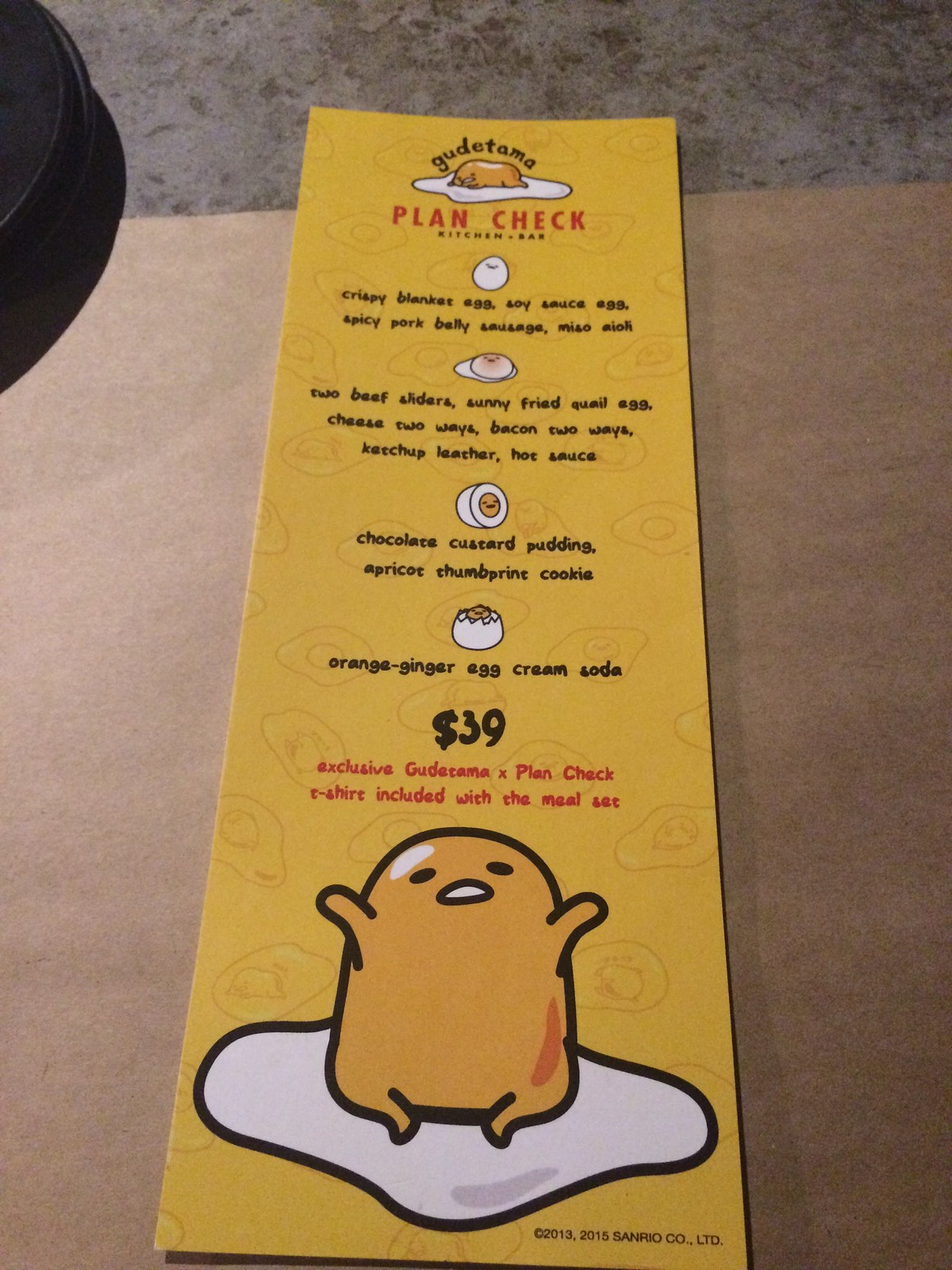This image showcases a menu themed around Gudetama, the lovable anthropomorphic egg yolk character from Sanrio. The menu, placed on a light brown table, is predominantly yellow with a background pattern of outlined eggs. There's a slight glimpse of what appears to be a plate in the top left-hand corner of the image.

The highlighted menu items include:

1. **Crispy Blanket Egg** 
2. **Soy Sauce Egg**
3. **Spicy Pork Belly Sausage**
4. **Miso Aioli**
5. **Two Beef Sliders**
   - Sunny-Fried Quail Egg
   - Cheese Two Ways
   - Bacon Two Ways
   - Ketchup
   - Leather Hot Sauce

For dessert, the choices listed are:
- **Chocolate Custard Pudding**
- **Apricot Thumbprint Cookie**

The beverage option includes:
- **Orange Ginger Egg Cream Soda**

It’s noted that the entire meal set is priced at $39 and includes an exclusive Gudetama Plan Check t-shirt. The menu title reads “Plan Check Kitchen + Bar.”

Overall, this descriptive caption vividly captures the essence of the Gudetama-themed menu, emphasizing its distinctive and playful food offerings along with the added merchandise incentive.